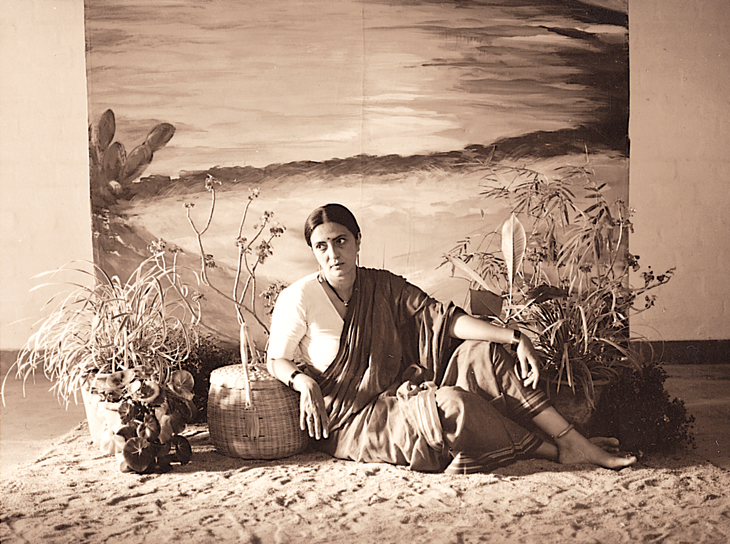This striking black-and-white photograph, with a sepia tone that adds a nostalgic quality, captures the serene image of an Indian woman adorned in traditional attire. She is comfortably seated on a sandy ground, resting her right arm on a wicker picnic basket, with her left knee drawn up and supported by her left arm. She is barefoot and wears a sari draped over her left shoulder, complemented by a bracelet and an anklet. 

Her gaze is thoughtfully directed over her right shoulder, adding a sense of contemplation to the scene. The intricate bindi (dot) between her eyes highlights her cultural heritage. Surrounding her are various dried plants and ferns that frame the composition elegantly, both on the ground beside her and in the backdrop. 

The backdrop itself is a painted, abstract scene with a watercolor texture, blending sunset hues and a grassy field, lending the setting an ethereal atmosphere. This flat wall with its impressionistic artwork suggests an indoor setting meticulously designed to evoke the outdoors. The details, from the traditional long skirt with its linear designs to the assortment of plants, collectively create an intimate and artistically enriched portrait.